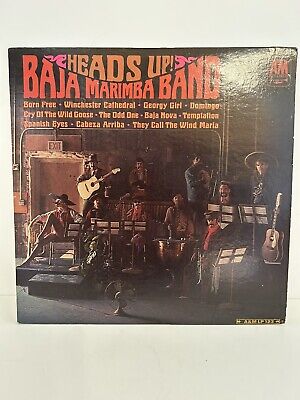The album cover for the Baja Marimba Band's "Heads Up" features ten men dressed in sombreros, presumably the band members. The men are arranged in two rows, with some holding acoustic guitars and others seated behind music stands, surrounded by various instruments. The setting appears to be a stage with a small fan on the floor in front of them and an exit sign visible above a door in the background. The album title "Heads Up" is prominently displayed across the top, with a distinctive artistic line running underneath. Below the title, "Baja Marimba Band" is written in large red letters. Further down, three lines of yellow text list the tracks included on the album: "Born Free," "Winchester Cathedral," "Georgie Girl," "Cry of the Wild Goose," "The Odd One," "Baja Nova," "Temptation," "Spanish Eyes," "Cabasa Arriba," and "They Call the Wind Maria." The cover stands upright against a light gray wall on a matching surface, with some glare visible at the top right corner of the image.